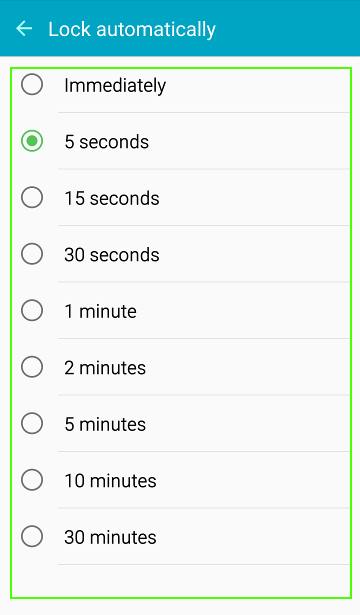In this image, we are looking at a screenshot of a settings menu. At the top of the screen, there is a teal-colored box with light blue text that reads "Lock automatically" and has a left-pointing arrow icon on the left side. Below the teal box, there is a white box outlined in green that lists various time intervals. The options begin with "Immediately" followed by "5 seconds," with the latter being marked by a green-highlighted circle, indicating it is selected. The list continues with "15 seconds," "30 seconds," "1 minute," "2 minutes," "5 minutes," "10 minutes," and "30 minutes." Each of these time intervals has a gray circle to its left, but only the "5 seconds" option is highlighted in green, showing it is the currently active selection.